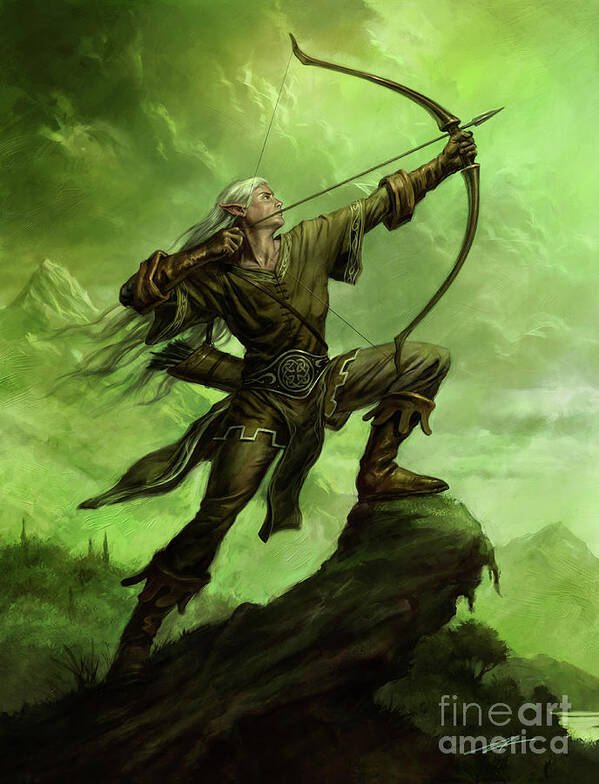The image is a detailed drawing of a man depicted in a superhero-style elven warrior pose, standing on an elevated, mossy rock. The entire scene is predominantly green, with varying shades from the sky to the distant mountains and the ground beneath him. The man has long, flowing platinum-colored hair and distinct elongated, pointy ears, typical of elven features. He is dressed in an all-in-one olive-green outfit, complete with a tunic, green leather gloves, pants, and boots. A quiver filled with arrows is strapped to his back. He has a bow in his hand, the bowstring pulled back, ready to release an arrow aimed at something above him. His striking young face, framed by his streaming hair, is set in a focused expression. The right side of the image is illuminated with white light, adding to the dynamic atmosphere of the artwork. The lower right corner bears the text "Fine Arts America."